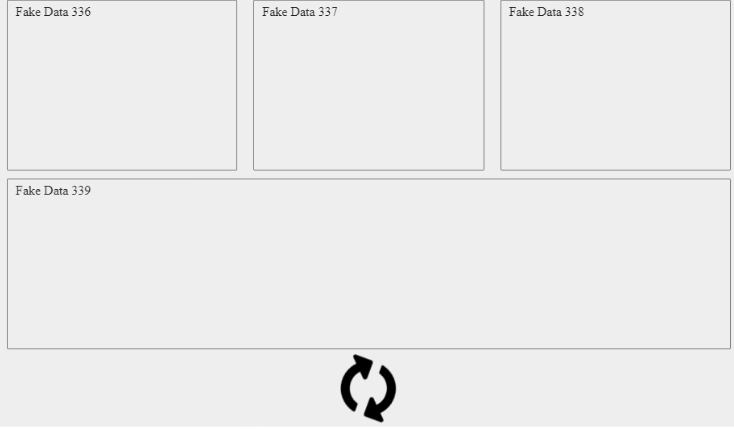The image features a light gray background with dark gray lines that form three squares at the top and one rectangle at the bottom. The top left square contains black text that reads "Fake Data 336," the middle square displays "Fake Data 337," and the right square shows "Fake Data 338." The rectangle at the bottom is labeled "Fake Data 339." At the bottom center of the image, two black arrows are curved into a circular shape, pointing clockwise. Additionally, a small portion of the gray background slightly protrudes from the left side of the dark gray line, though this detail is barely noticeable.